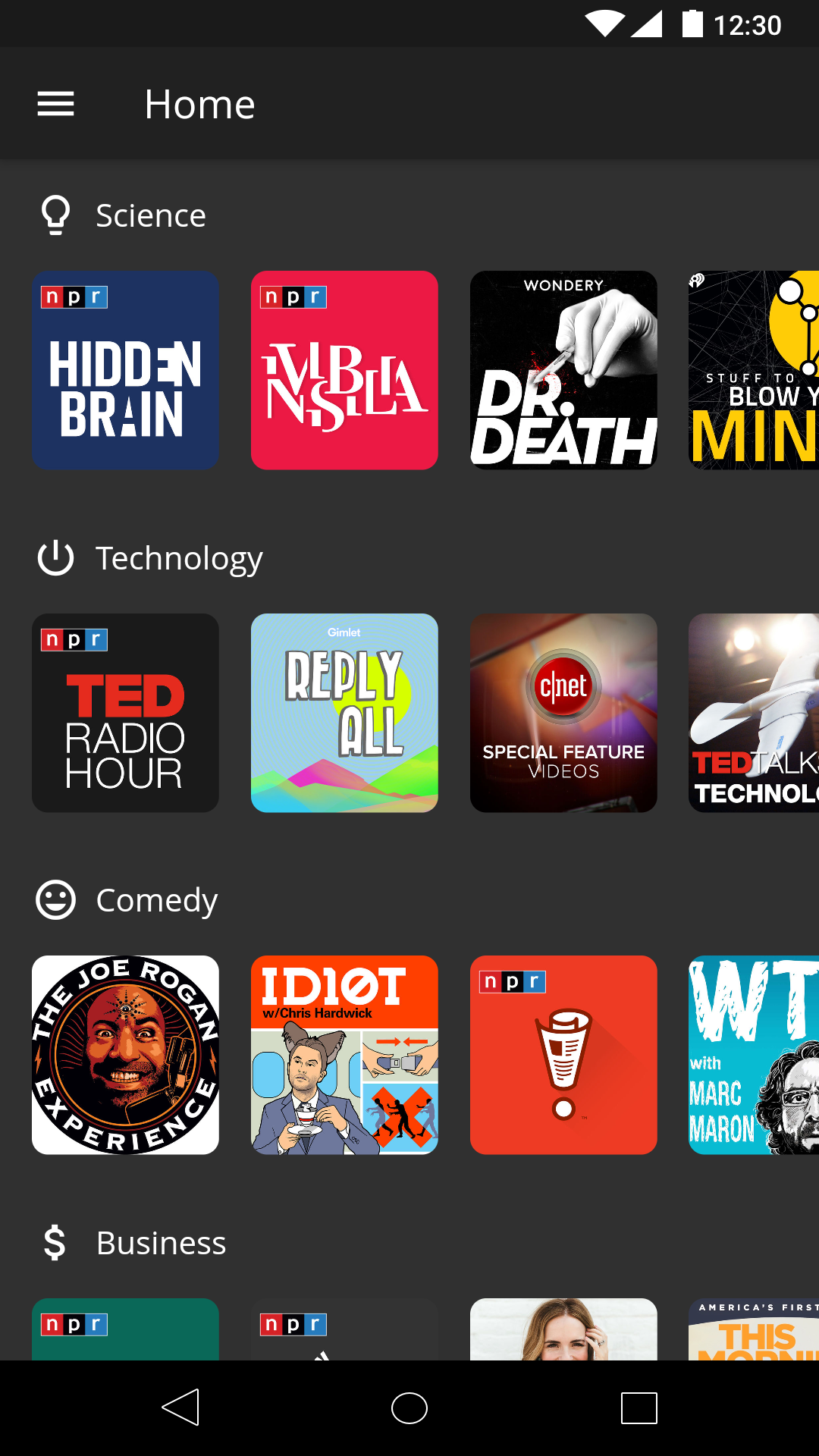The image depicts a smartphone screen displaying rows of podcasts. At the top right corner of the screen, various status icons are visible, including the Wi-Fi signal, cellular connection, and a fully charged battery, alongside the time, which is 12:30. These items appear on a black background. On the left side of the screen, there's a vertical tab menu featuring the "Home" option. The majority of the remaining background is gray. 

In this tab menu, podcasts are categorized into four sections: "Science," "Technology," "Comedy," and "Business," listed from top to bottom. Each category shows rows of podcasts arranged horizontally. Each row features four square-shaped podcast icons, each with its own unique name and design displayed in white text. 

At the very bottom of the screen, there are three navigation icons outlined in white on a black background. From left to right, they include a back arrow (sideways triangle), a home button (circle), and a recent apps button (square). These navigation icons complete the design of the smartphone interface.